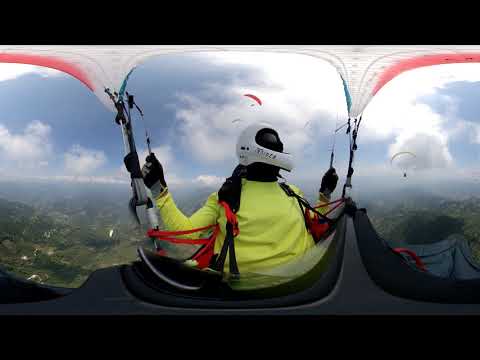The image depicts a person in mid-air, seemingly about to jump or currently skydiving from a helicopter or similar aircraft. The focus is on their back, clad in a bright yellow long-sleeved jacket, with a striking white helmet and black gloves. They are positioned in the open doorway or near the edge of the craft, with a clear view of the ground below. The interior of the vehicle features a black bottom and white top. Outside, the scene unfolds with rolling green hills dotted with small white houses, extending into a vast, partly cloudy blue sky. The overall impression suggests a thrilling moment amidst picturesque surroundings, blending the excitement of high-altitude adventure with the serene beauty of the landscape below.